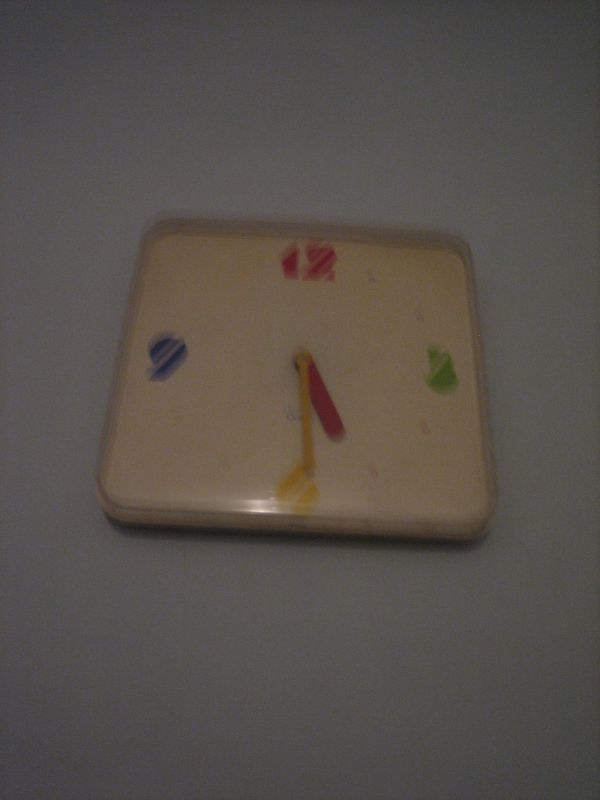The photograph portrays a square-shaped kids' wall clock with a creamy white clock face and a white plastic border. The background is solid gray and blurry, due to the low-quality camera used to capture the image. The clock is designed with only four numerals: a red 12 at the top, a green 3 on the right, a yellow 6 at the bottom, and a blue 9 on the left. The remaining positions are marked by light-colored dots. The clock has an analog display with a red hour hand and a yellow minute hand, indicating the time is approximately 5:30. The clock face appears to be covered by a clear protective case, and there is light reflecting off its surface.